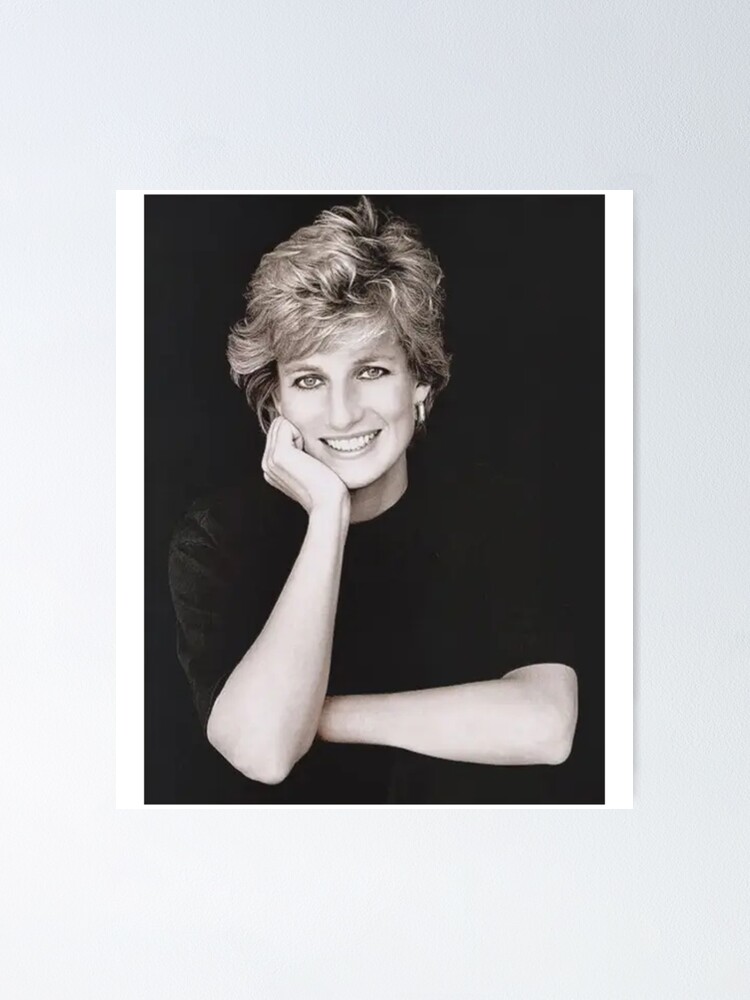This image features a black and white portrait of Princess Diana, taken possibly during the early 1990s when she was in her 30s. In this striking photograph, Princess Diana's short, light hair elegantly frames her face, with soft curls and bangs. Her eyes, adorned with a touch of mascara and eyeliner, gaze directly into the camera, lending an intimate and soulful connection. 

She is adorned with a delicate earring in her left ear and a dark shirt that contrasts with the black backdrop. The photo captures her classic, radiant smile that reveals her white teeth, further emphasized by her light makeup. Princess Diana's right cheek gently rests on her right hand, with her elbow supported on a surface, creating a serene and approachable pose. The entire image, bordered in white, is placed against a grey surface, enhancing the timeless elegance and grace of the late Princess of Wales.